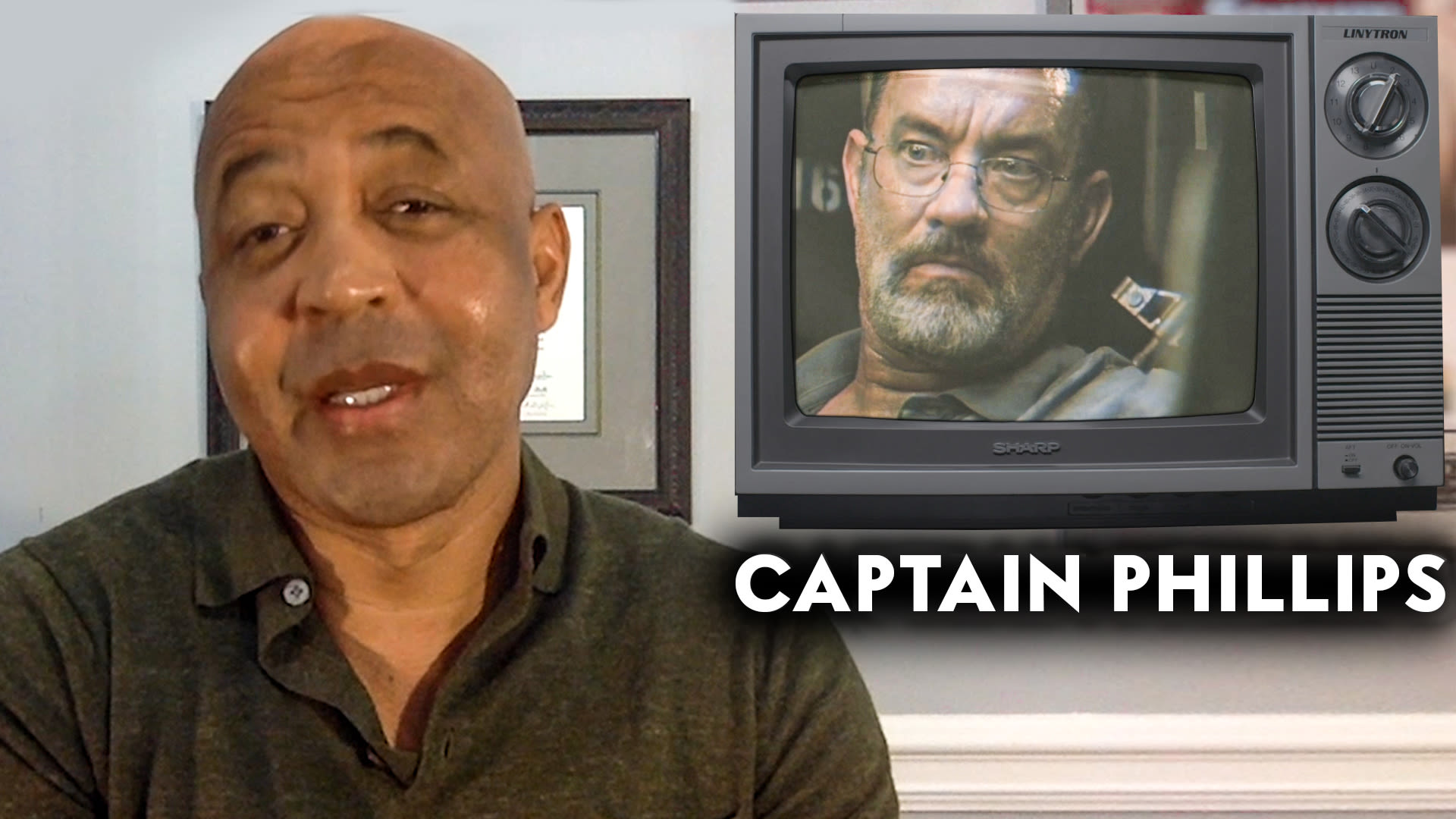The rectangular photograph captures a scene with two focal points: an African-American man in the foreground and an old-style television set in the background. The man, wearing a collared shirt that appears to be dark green or gray, is facing forward, possibly mid-conversation or reviewing a movie. Covering part of a framed picture or certificate on the wall behind him, his figure is set against a gray background with a piece of white baseboard visible at the bottom right.

In the upper right corner of the image, an antiquated, boxy TV set—marked "Linetron" with two knobs on the right—is prominently displayed. The TV screen shows a man who closely resembles Tom Hanks in his role from the movie "Captain Phillips," identified by the white lettering underneath. Hanks appears with a graying, close-cut beard and glasses, sporting an angry or bewildered expression. The intricate details encapsulate both modern and nostalgic elements, merging the man's present-day interaction with the historical feel of the vintage television.